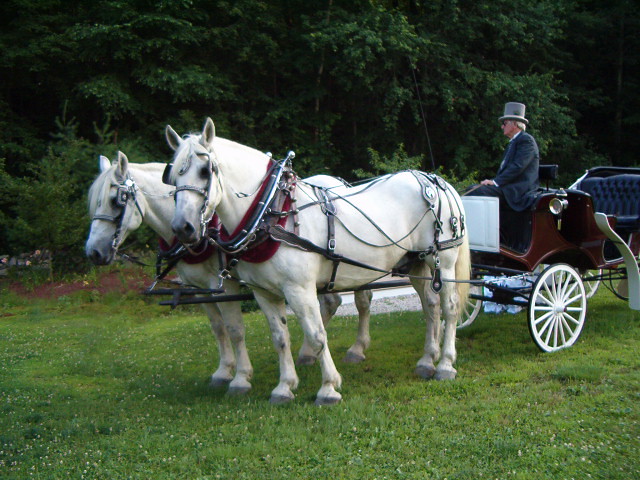This full-color horizontal-rectangular image captures a horse-drawn carriage in a lush, green park during the daytime. The main focus is a pair of white horses, adorned with a decorative yoke and harnesses, pulling a two-wheeled brown carriage with white wooden wheels. The carriage features padded blue seats and at least one light for night-time riding. Seated in the driver’s seat is a man wearing a gray top hat and a long, formal coat. His hands are positioned as if holding the reins. The background reveals a serene scene of trees and a verdant field of grass, enriching the outdoor setting.